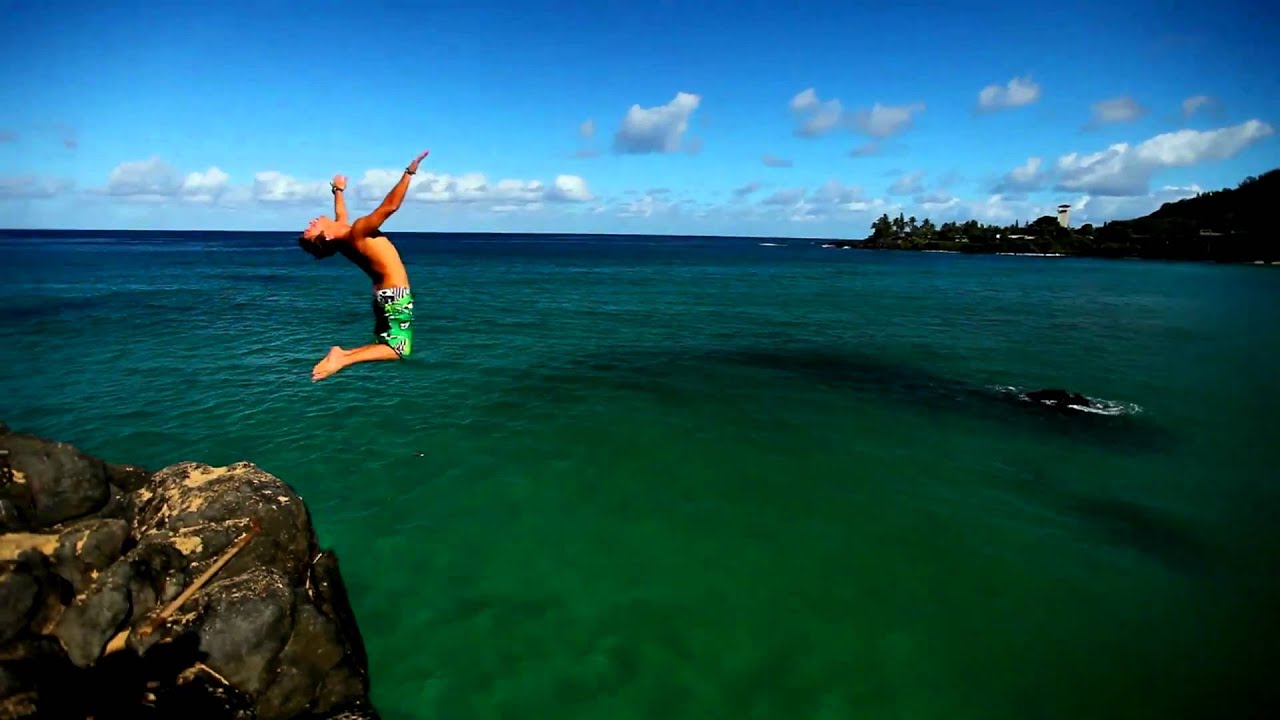In the image, a young man, appearing to be in his early 20s, is captured mid-jump from a rock cliff into the ocean. His green, black, and white swim shorts contrast with the varying shades of green and blue in the water below. Both his arms are outstretched, adorned with a watch and bracelets, while his head is tilted back and his legs are tucked behind him, hinting at a possible backflip. The cliff he has jumped from is sizable but not excessively high and is surrounded by an array of gray and brown rocks. To the left of the image, more rocks protrude from the water. In the distance, an empty boat floats on the water, and further ashore, there are groups of trees, rolling hills, and a prominent large tower. The sky is dotted with clouds, completing this dynamic outdoor scene.